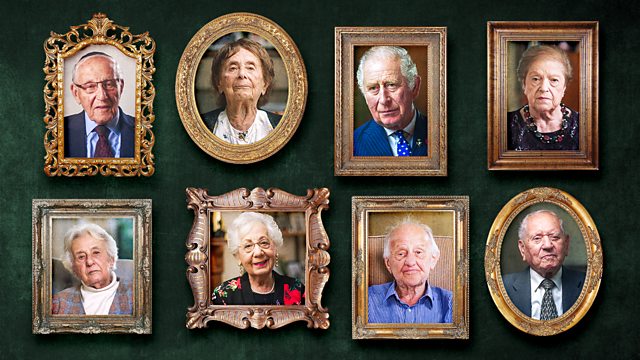The photograph captures a carefully arranged series of eight framed portraits of elderly individuals, hanging on a dark green wall in two rows of four. Each portrait is encased in a decorative frame, ranging from rectangular and square shapes to more ornate and oval designs, predominantly in gold. The subjects appear to be a random mix of four women and four men, all generally facing the camera.

In the top row, the first portrait in a square frame depicts an elderly man with glasses, a blue suit jacket, light blue collared shirt, dark necktie, and a yarmulke. Next, in a round brass frame, an elderly woman in a white blouse with dark shoulders looks directly at the viewer. The third portrait, in a square frame, features King Charles in a blue suit jacket, white collared shirt, and blue tie. The final portrait of this row is a rectangular frame showcasing a late middle-aged woman also staring at the camera.

The second row starts with a square frame containing an elderly individual with short white hair, wearing a patterned vest and a white turtleneck. Next, a smiling elderly woman with glasses and red lipstick appears in a rectangular frame, adorned in a black floral-patterned jacket. The following square frame features a man in his late 70s with sparse white hair and a blue button-down shirt, showing a slight smile. The last oval brass frame of the row presents an unsmiling elderly man in a gray suit jacket, white collared shirt, and a patterned dark necktie. Excluding King Charles, the rest of the individuals remain unrecognizable.